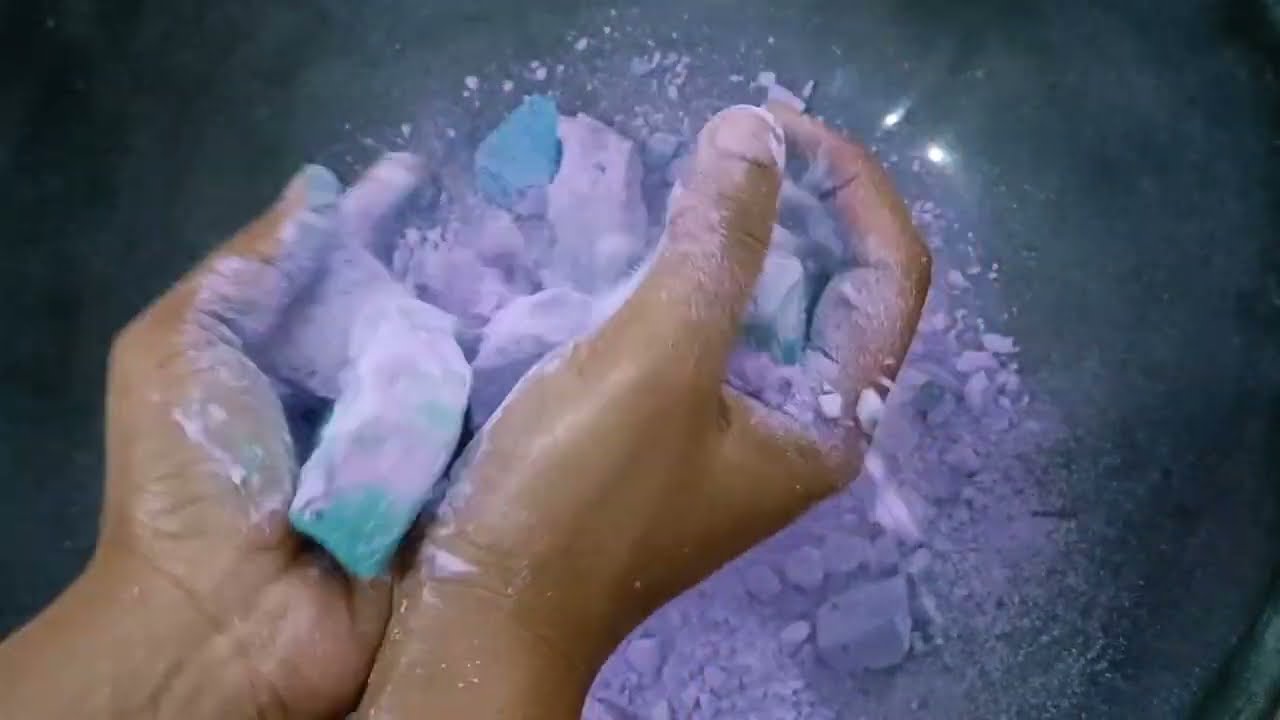A close-up photo captures a pair of tan-colored hands, holding and crushing blocks of chalky purple and teal blue material. The chalk, which appears almost talc-like, is breaking apart and falling through the fingers onto a turquoise surface below. The hands are covered with residue from the chalk, highlighting both the powdery consistency and vibrant colors of the material. Chunks and small pieces of the chalk can be seen scattered on the surface, suggesting that the material is quite fragile and crumbling easily as it is manipulated. The background and overall setting, possibly outdoors, underscore the hands as they work to break apart the colorful chalk.